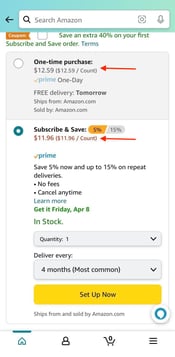A screenshot of the Amazon website shows a user in the process of purchasing an item through the Subscribe & Save program. The page displays two purchasing options: a one-time purchase or the Subscribe & Save option that offers recurring deliveries at a discount. The user has chosen the Subscribe & Save option, receiving a 5% discount, reducing the price from $12.59 to $11.96. Additional text indicates that users can save up to 15% on repeat deliveries with no fees, with the option to cancel anytime. The item is available for delivery by Friday, April 8th, and the user has selected a delivery frequency of every 4 months, although this can be adjusted via a dropdown menu. There is a prominent yellow button labeled "Set up now." At the bottom of the screen, there are icons for the homepage, personal account, an empty shopping cart, and a hamburger menu for additional options.